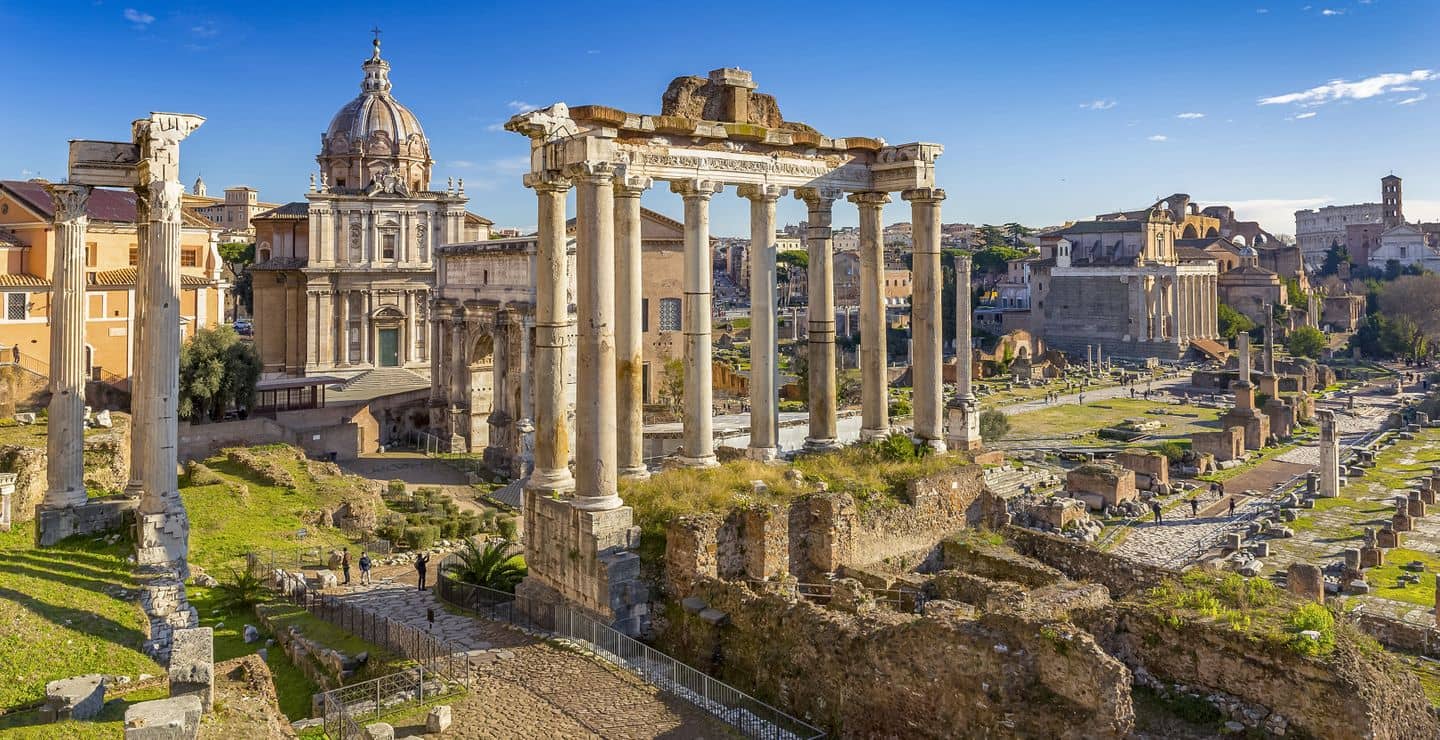This photograph captures the sprawling ruins of an ancient Roman city juxtaposed with its modern-day surroundings. Dominated by towering white columns and intricate, crumbled architecture, the scene stretches into the distance, where the iconic outline of the Roman Colosseum can be spotted to the right. Among the ancient structures are remnants of walls and what appear to be crypts, creating a contrast between the historical and the contemporary. An ornate building with a dome, possibly a cathedral, stands prominently, displaying detailed craftsmanship. Some columns remain upright amidst the ruins, covered in patches of grass and moss, while people on the ground appear tiny in comparison, emphasizing the monumental scale of the ancient structures. The scene is bathed in beautiful weather with a bright blue, mostly cloudless sky, adding to the grandeur of this historical juxtaposition.